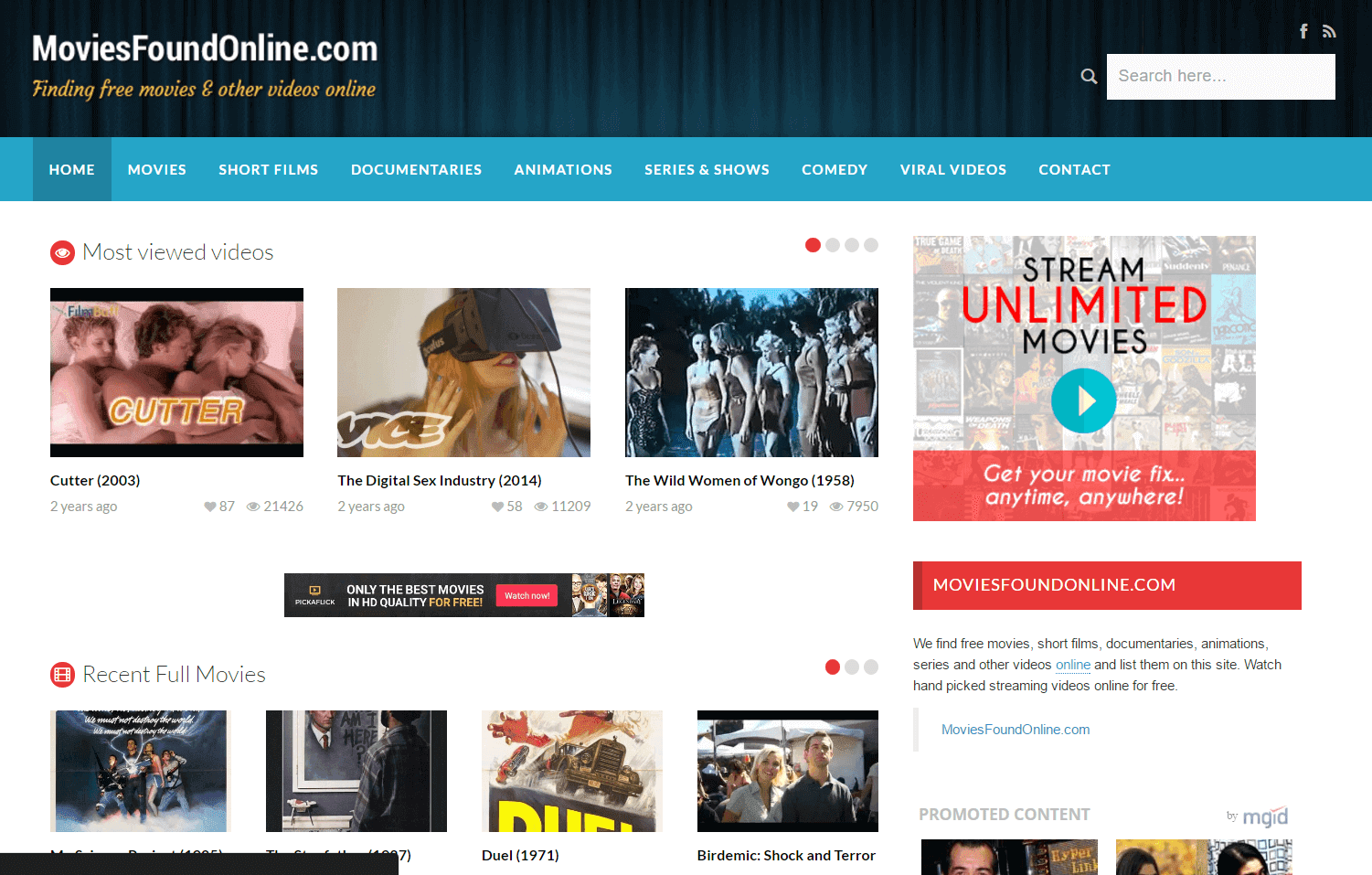The web page for MoviesFoundOnline.com is efficiently designed to help users find free movies and other videos. To the right is a search bar labeled "Search here," situated below a Facebook logo and a Wi-Fi icon. Beneath these elements, a navigation menu includes tabs for Home, Movies, Short Films, Documentaries, Animations, Series and Shows, Comedy, Viral Videos, and Contact.

Below the navigation menu is a section titled "Most Viewed Videos," featuring three entries with their respective details and an indication of three additional pages. The first video is "Cutter" (2003), uploaded two years ago with 87 likes and 21,426 views. The second is "The Digital Sex Industry" (2014), uploaded two years ago with 58 likes and 11,209 views. The third entry, "The Wild Women of Wongo" (1958), also uploaded two years ago, has accrued 19 likes and 7,950 views.

Further down is the "Recent Full Movies" section, where the first two titles are obscured. Visible entries include "Duel" (1971), an excellent movie, alongside "Birdemic: Shock and Terror." This section also indicates the presence of two additional pages.

On the right side, an advertisement promotes unlimited movie streaming with the slogan, "Stream Unlimited Movies, get your movie fix anytime, anywhere!" Reinforcing the website's purpose, a text blurb affirms, "Moviesfoundonline.com – We find movies, short films, documentaries, animation series, and other videos online and list them on this site. Watch handpicked streaming videos online for free." Below this is a section for promoted content.